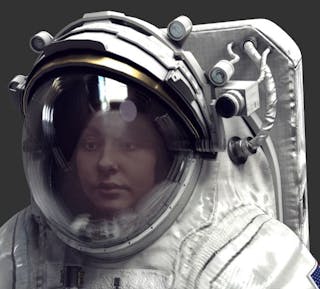This image captures a person clad in a detailed white spacesuit, cropped from their lower chest up to the top of their helmet. The spacesuit features a white fabric with visible pleats and seams, while a small, partially visible patch—possibly the corner of the American flag—is located on the shoulder. The helmet, globe-like and made of a clear glass pane, fully encompasses the wearer's head and is bordered by a golden frame. The person's face is visible through the visor, displaying a neutral expression with closed mouth and forward-looking eyes, although details about their hair color remain obscured by darkness above their forehead. Three knobs can be seen in the upper right section of the helmet, hinting at adjustable functionality. The helmet seems equipped with multiple protective shields that can be lowered over the face, ensuring added layers of defense in space. A reflection is noticeable on the helmet's glass surface, indicating its transparency and the ambient lighting. Attached to the person's back is a rectangular backpack featuring numerous tubes and hoses connected both to the pack and the suit, suggesting a life-support or environmental control system. This backpack also contains various gauges and possibly a small camera and light above the left shoulder. The overall background of the image is slightly dark, further accentuating the illuminated and intricate design of the space suit and helmet.